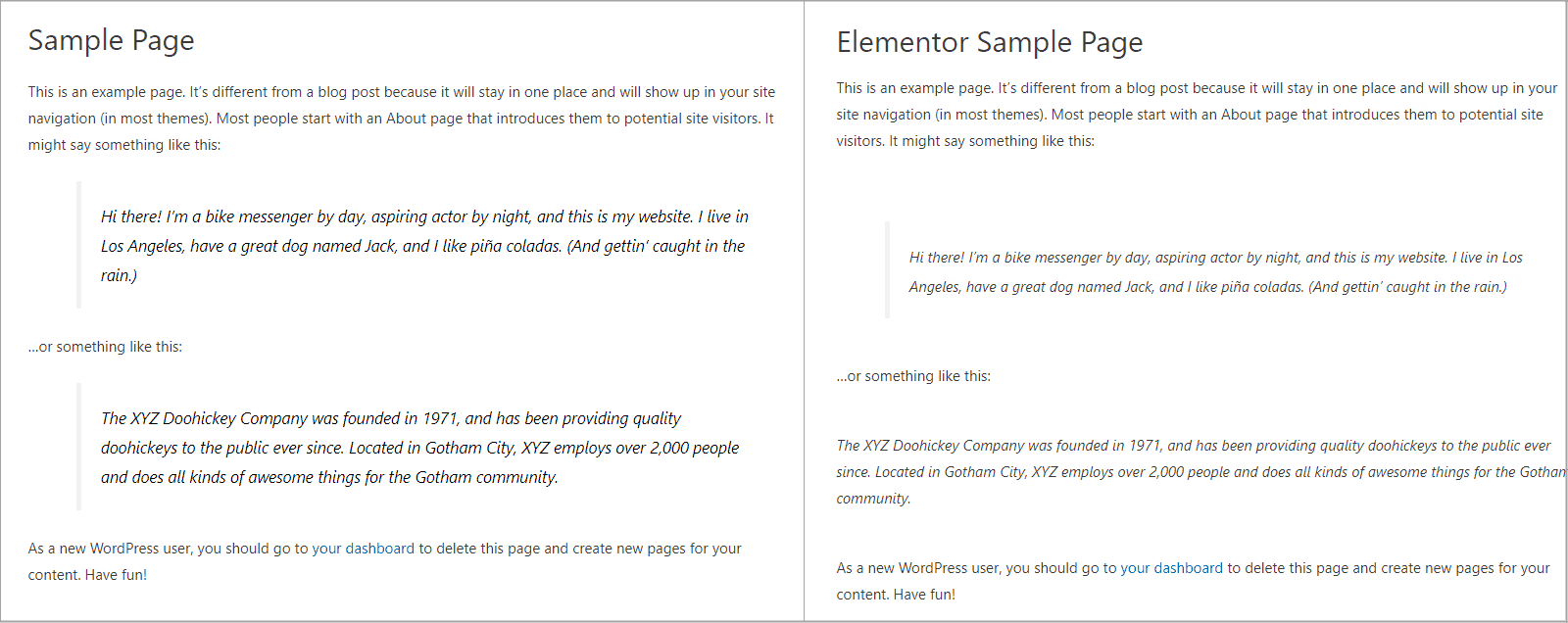**Detailed Caption:**

The image is a screenshot of a sample page designed to demonstrate an example blog post for the WordPress website. This introductory page is intended for users who are preparing to create their first blog post. 

The screenshot features a very simplistic layout, consisting of two boxes, each outlined in gray. The box on the left is titled "Sample Page." Beneath this title, the text explains that the page serves as an example and differs from a blog post by remaining stationary and appearing in site navigation across most themes. It advises new users to start with an "About" page that introduces them to potential site visitors. A suggested template for this introduction might say, "Hi there, I'm a bike messenger by day, aspiring actor by night, and this is my website. I live in Los Angeles, have a great dog named Jack, and I like pina coladas and getting caught in the rain..." Alternatively, it might provide a business-oriented example like, "The XYZ Doohickey Company was founded in 1971 and has been providing quality doohickeys to the public ever since. Located in Gotham City, XYZ employs over 2,000 people and does all kinds of awesome things for the Gotham community." The page then recommends new WordPress users visit their dashboard to delete this sample page and create new content for their site.

The box on the right contains identical information but is translated into Spanish, ensuring accessibility for Spanish-speaking users.